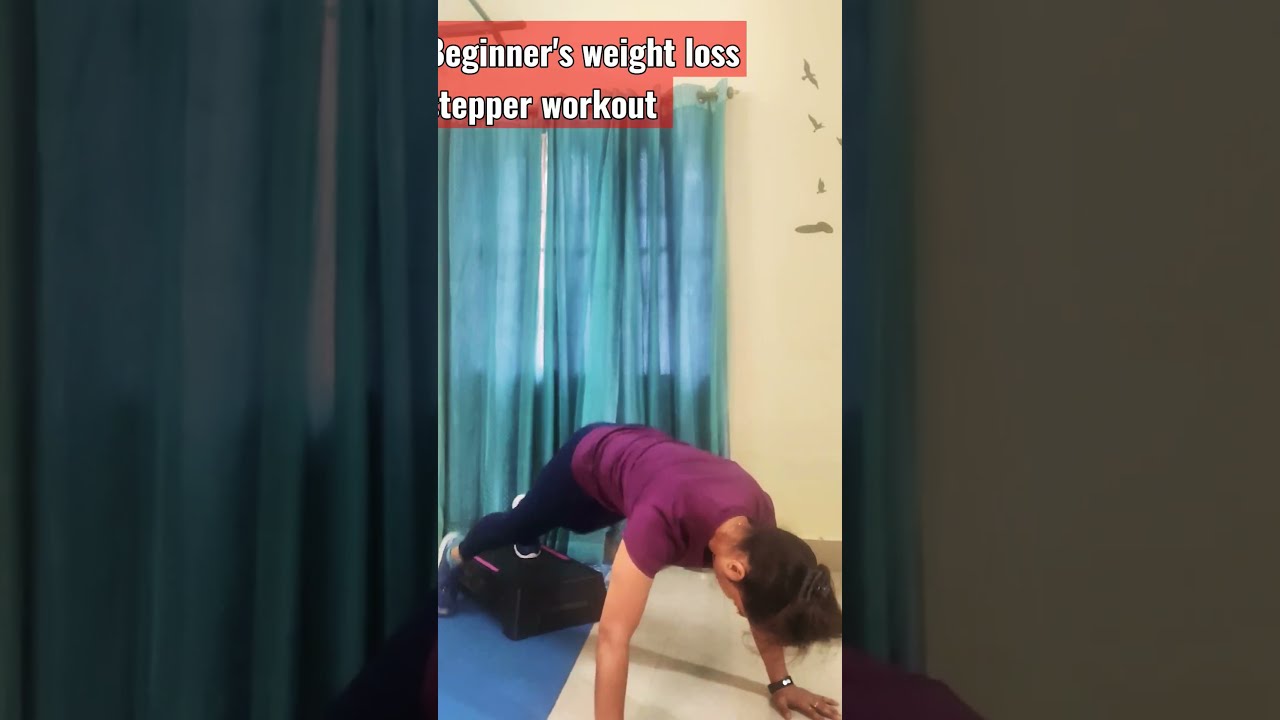A vertically taken cell phone image showcases a woman in the midst of her workout, with her facing downward in a plank position. She is wearing a purple workout t-shirt and black leggings, sporting a smartwatch or fitness watch on her left wrist. Her dark brown hair is tied up in a ponytail, hanging down as she supports her weight with her hands on the ground. One of her feet is placed on a black stepper while the other foot remains on a white-tiled portion of the floor. The room features light blue curtains that cover a window in the background, and the floor transitions from a blue carpet on one side to a white material on the other. The walls are white with a few stenciled birds visible on the right-hand side. At the top of the image, a red box with white lettering reads, "Beginner's Weight Loss Stepper Workout," suggesting that the woman is demonstrating an exercise routine for a possible workout video.